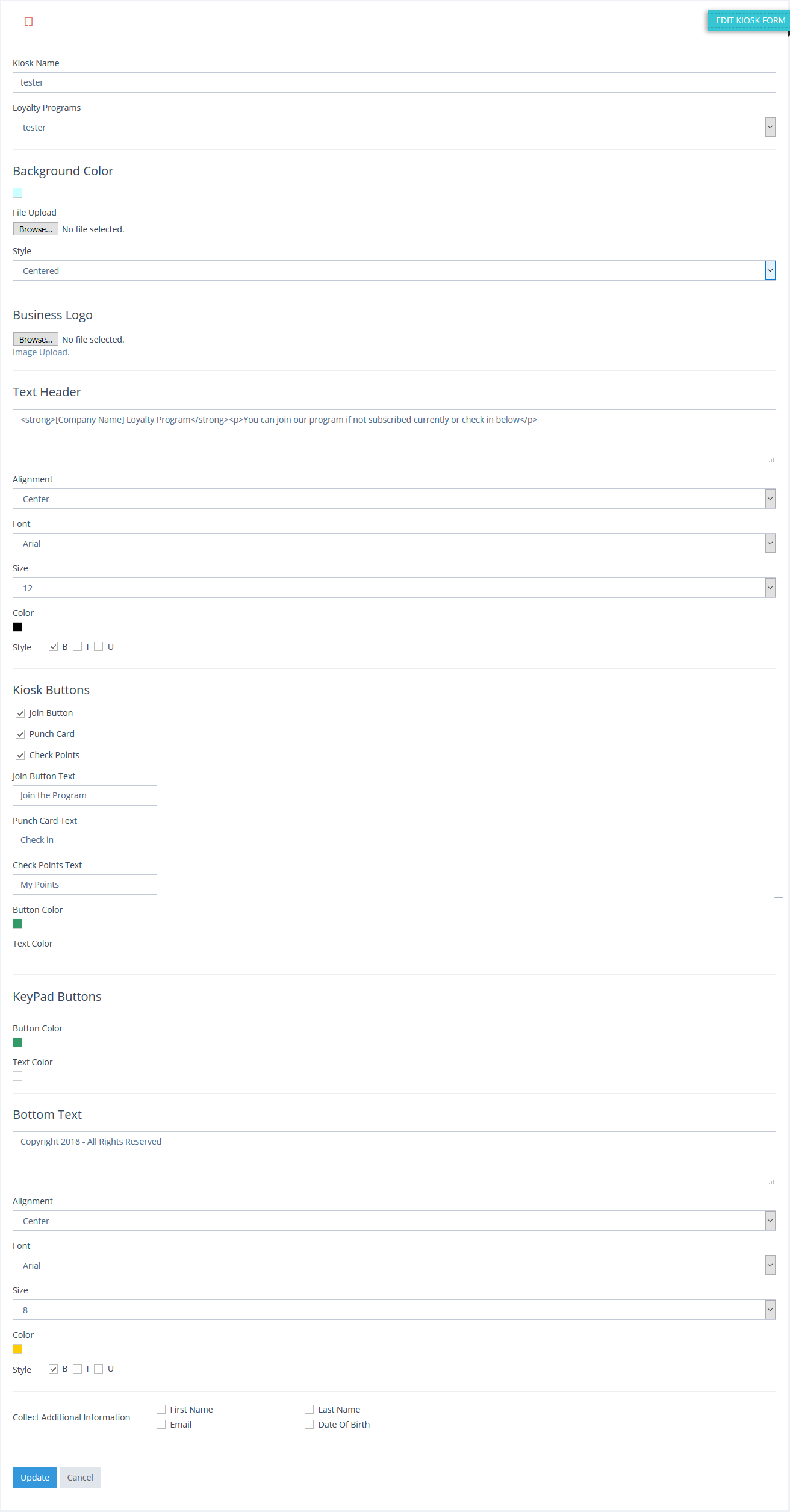This image appears to be a screenshot taken from a software interface on a computer or phone, characterized by extremely tiny, hard-to-read text that becomes even more blurry when zoomed in. In the upper right corner, there is a teal rectangular shape. At the top of the interface, there are two items with drop-down menus. Below that, a section labeled "Background Color" features another drop-down menu.

Next, there is a heading titled "Business Logo," followed by a "Text Header" section containing a text input box. Under the "Text Header," there are three more drop-down menus. The subsequent heading "Kiosk Buttons" includes three pre-selected choices.

Further down the interface is the "Keypad Buttons" section, which contains a bottom text heading with a text input box underneath. This is followed by an additional three drop-down menus. In the bottom-left corner, there are two buttons: the first is blue, possibly labeled "Submit," and the second is gray, possibly labeled "Cancel."